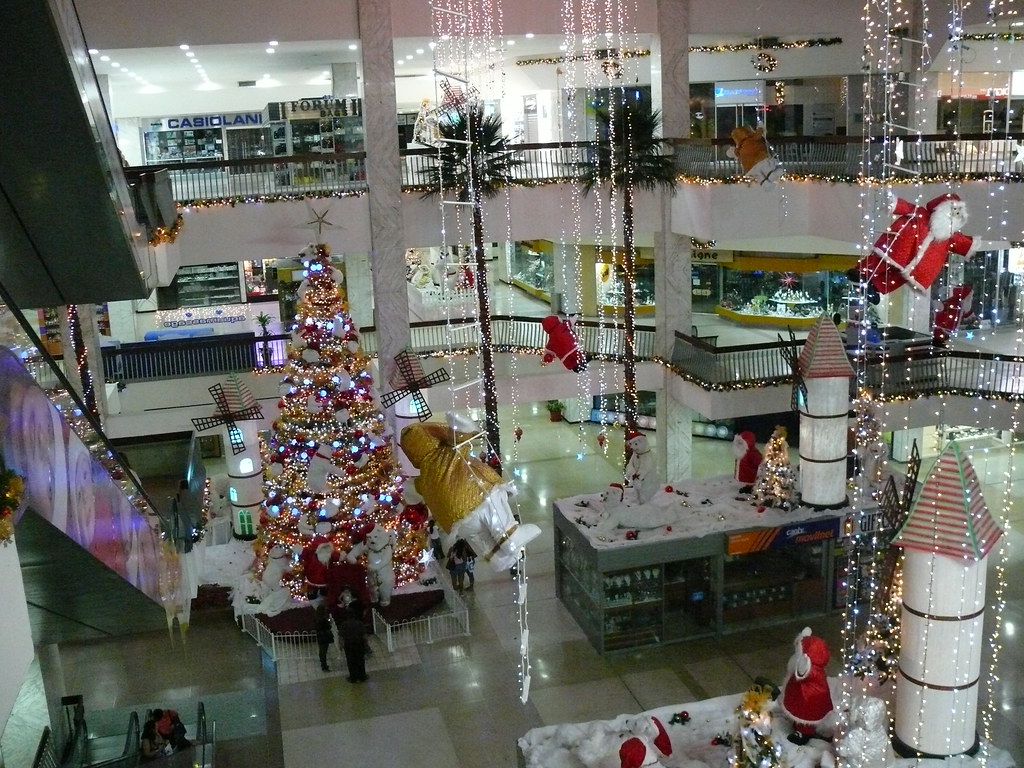The photo depicts the festive interior of a multi-level mall during Christmas time. The perspective is from an upper floor, likely the second or third level, looking down into a spacious atrium. The floor below features a shiny beige and white pattern with square tiles, creating a polished look. Dominating the scene is a grand Christmas tree adorned with gold, white, and hints of green and red ornaments positioned to the left. In the vicinity are staircases leading to various levels, enhancing the sense of verticality in the space. Festive Santa figures dangle from Christmas lights descending from an unseen high ceiling. Visible in the background are railings of an upper floor, suggesting multiple shopping levels, and various shop entrances that animate the bustling holiday atmosphere. Scattered smaller decorated Christmas trees and cashier stations contribute to the vibrant, festive setting.